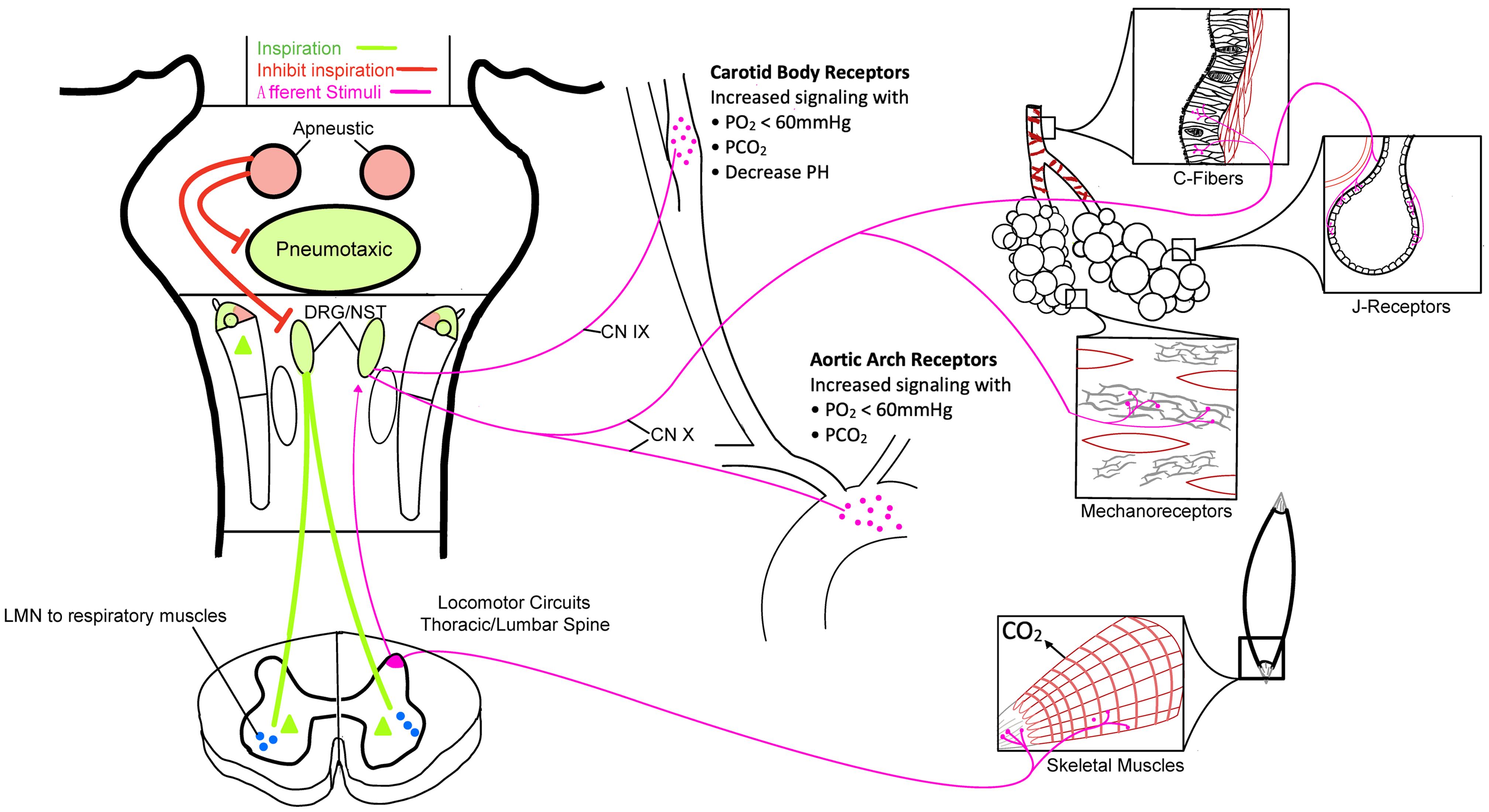This image is a detailed diagram of the human body's nervous and muscular systems, focusing on the interaction between spinal columns, skeletal muscles, and respiratory function, particularly in the context of paralysis. Central to the diagram is the thoracic lumbar spine, with labeled components such as "locomotor circuits" and "LMN to respiratory muscles." The chart also highlights various receptors and fibers, including the carotid body and aortic arch receptors, and features diverse colors for differentiation: green lines indicate "inspiration," orange lines denote "inhibit inspiration," and pink lines represent "afferent stimuli." This intricate layout illustrates how pressure from the spine on nerves can impact respiratory muscles, potentially inhibiting critical receptors and thus affecting lung function. The overall color scheme of the diagram includes purple, black, and white, tying together the various elements of this complex physiological interaction.